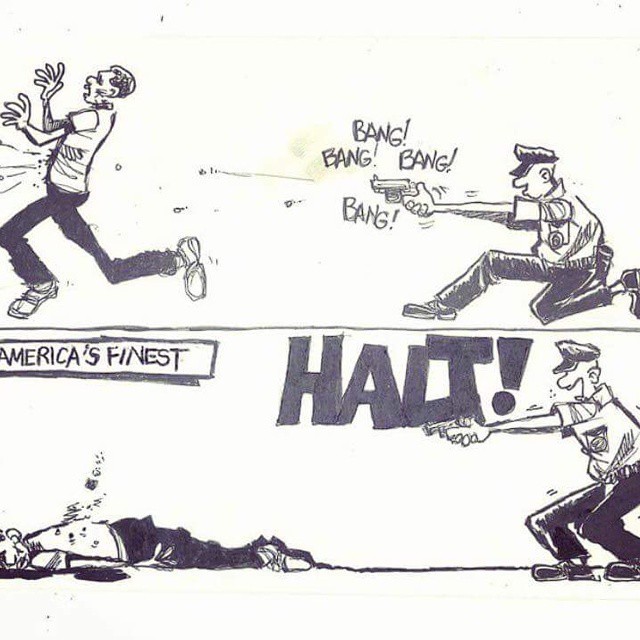The image is a black and white cartoon drawn on white paper, depicting two scenes divided horizontally. In the top half, a policeman is kneeling down on the right side, aiming a gun that releases the words "bang bang bang" as he fires. To the left, an African-American man is seen running away in fear with visible bullet trajectories heading towards him. In the bottom half, the scene shifts; the policeman is now standing in a crouched position still holding the gun and shouting "HALT" in large capital letters. The man who was running is now lying on the ground, seemingly lifeless, with a sign nearby reading "America's Finest." The cartoon appears to critique the American police system, particularly its tendency towards excessive use of force against African-Americans, capturing a politically charged and ironic commentary on current social issues.